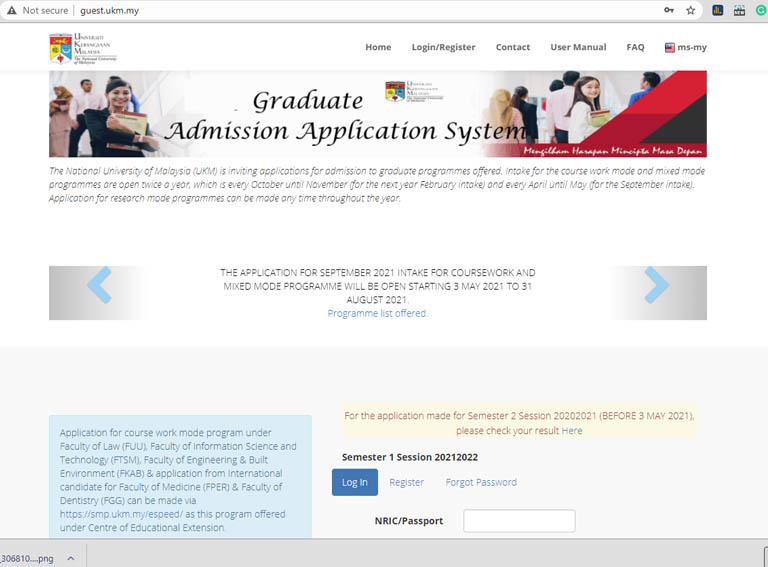The image appears to be a screenshot of a web page from the admission portal of the National University of Malaysia (UKM). 

At the top of the page, there is a search bar accompanied by a triangular icon with an exclamation mark indicating "Not secure" followed by "guest.ukm.my." To the right of the search bar, there are a key icon, a star icon, and further right, three more icons: a chart, a new item, and a green circle with an arrow forming a loop.

Below this bar, the university’s shield logo is displayed, which features a red bar at the top and is divided into three sections (yellow, blue, and white) at the bottom. To the right of the logo, navigation headers include "Home," "Login/Registration," "Contact," "User Manual," "FAQ," and "ms.my."

The main content area features a large heading that reads "Graduate Admission Application System." Below this heading, there is a picture of students on a staircase holding books, and another photo to the right shows students walking away with one looking back towards the camera.

The text below these images provides information about the National University of Malaysia and its invitation for graduate admissions. It specifies that the application period for the September 2011 intake for coursework and mixed-mode programs will be open from May 3rd, 2021, to August 31st, 2021. Blue arrows on either side of this text allow for navigation.

Below this section, within a blue text box, additional information is displayed alongside buttons labeled "Login," "Register," and "Forgot Password." Finally, at the very bottom of the page, there is a gray bar running across the width of the screen.